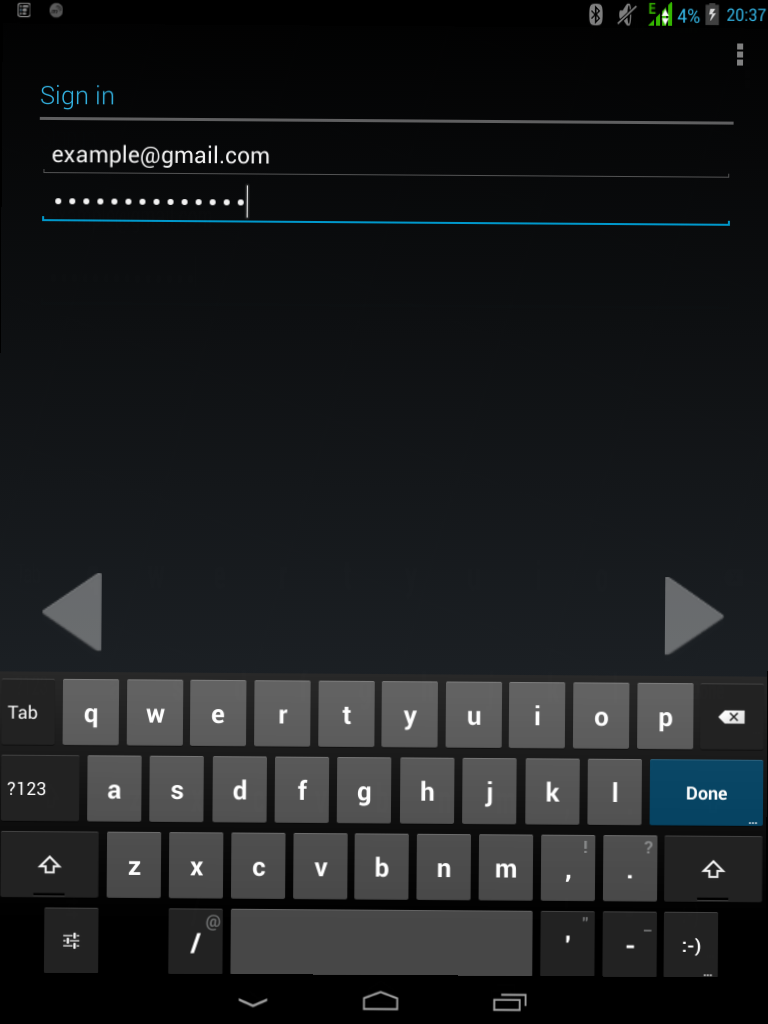A phone screenshot with a black background showcases a sign-in interface. At the top right of the screen, a Wi-Fi signal icon is visible along with a nearly depleted battery indicator at 4%. The topmost line of the interface reads "Sign in" in blue text, followed by "example@gmail.com" just below it. A series of dots, representing hidden characters in a password field, is shown underneath the email address. The majority of the screen remains blank and black, drawing attention to the keyboard at the bottom. The QWERTY keyboard encompasses most of the lower part of the display and is currently active for input. On the far right of the dot sequence, the blinking cursor indicates that the user is still typing. The top row of the keyboard features left and right arrow icons. At the very bottom, a black border houses a down arrow, a home icon, and a "more" tab icon, which likely provide quick access to additional navigation options.